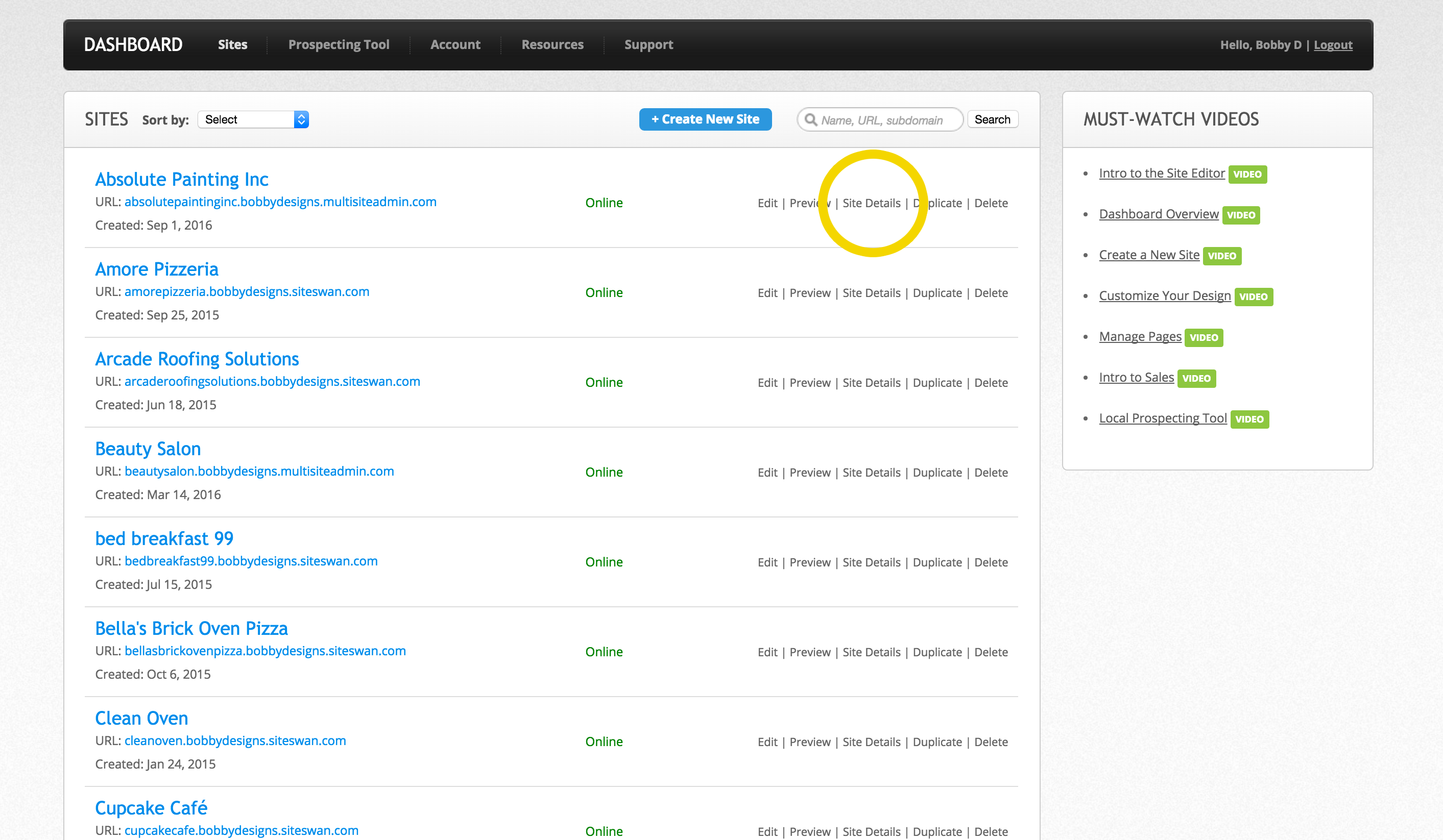On this web page with a light gray background, the top section features a black header with capitalized white lettering that reads "Dashboard." To the right of the header, a menu follows. The first menu option, "Sites," is displayed in small white lettering. Subsequent menu items transition to gray and include "Prospecting Tool," "Account," "Resources," and "Support."

Below the header, a light gray sub-header spells out "SITES" in medium gray capital letters. Adjacent to this, in smaller black lettering, it reads "Sort by:" followed by a dropdown menu labeled "Select." A long blue rectangular icon with white writing and a plus symbol states "Create New Site."

Further to the right, an oval-shaped search bar allows for query entry, marked by a gray magnifying glass icon on the left. Inside the bar, italicized text provides guidance: "Name, URL, Sub domain." The search function is completed with a button on the right, featuring black lettering encased in a black border.

On the far right, another light gray header displays "MUST-WATCH VIDEOS" in dark gray or black capital letters. Below this header lies a white rectangular background area housing a bulleted list of clickable links. Each link is paired with a green rectangular shape labeled "Video" in white letters. The options listed include "Intro to the Site Editor," "Dashboard Overview," "Create a New Site," "Customize Your Design," "Manage Pages," and "Intro to Sales and Local Prospecting Tool."